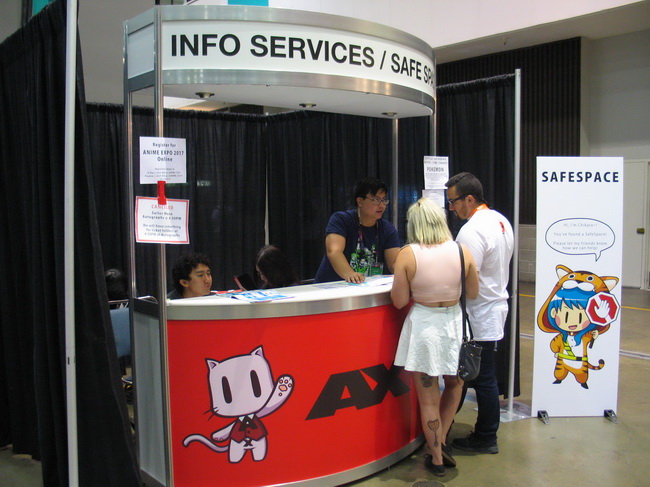The photograph captures an information desk prominently labeled "Info Services / Safe Space" on a white plastic sign with gray trim and black uppercase font. The red front panel of the desk features an illustration resembling Hello Kitty and the letters "AX." Behind the desk, two Asian men are present—one standing and talking to a couple at the counter, and the other seated. The standing man is wearing a blue t-shirt and glasses. The couple is identified as a Caucasian man and woman; the woman has blonde hair, wears a pink sleeveless top and white skirt, and has a heart tattoo on her left calf, while the man wears a white top, black pants, and glasses. To the right of the desk, a white vertical sign displays "Safe Space" and a cartoon character with blue hair in a tiger costume holding a stop sign. The background appears to be a generic mall setting with gray concrete floors and white walls. Additional signs posted on the support of the main sign include one that reads "Anime Expo 2017." A woman with long hair is faintly visible in the background, partially obscured by the desk. The booth itself also has a black curtain around its rear.